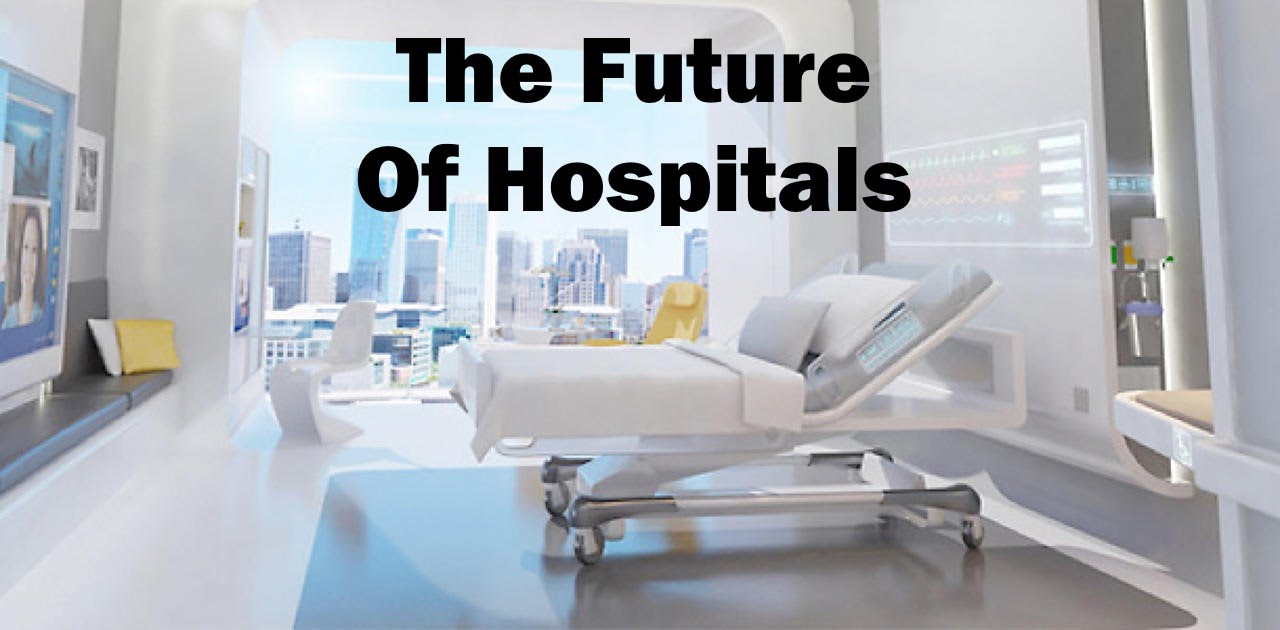The advertisement, bearing the phrase "The Future of Hospitals" in bold black lettering, showcases a sleek, modern hospital room. At its center is an innovative, contemporary hospital bed, notably slimmer than traditional models and devoid of any cords. The bed, partially propped up, draped in white linen with gray sheets, includes a large white pillow and a smaller gray pillow. The bed is situated atop a gray mat on a pristine white floor. To the left are comfortable seating options: a bench adorned with a yellow pillow and a white pillow, and a white chair positioned a few feet away. The room exudes a futuristic ambiance, emphasized by a large window that frames a silhouetted cityscape of tall buildings. The walls, free from clutter, feature a high-tech display system projecting vital signs, replacing the need for multiple machines. Overall, this immaculate environment, with its sleek design and advanced technology, epitomizes the future of hospital care.